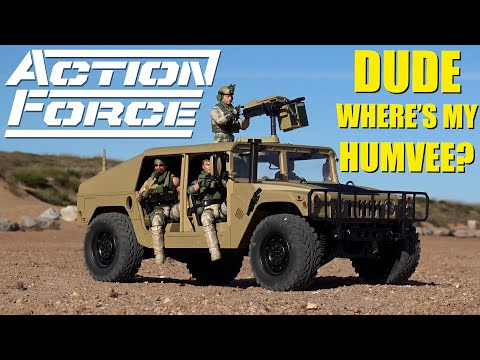The image depicts a dark olive-green military Humvee, likely an advertisement for children's action figures labeled "Action Force." The scene features three soldier figures, dressed in army attire, in a barren, rocky desert field under a blue sky. One soldier is seated in the back seat with a leg hanging out, while another is in the passenger seat, also with a leg outside the vehicle due to the absence of doors. A third soldier is positioned on top of the vehicle, manning a mounted gun turret. The image includes white text stating "Action Force" on the top left and yellow text on the top right that humorously reads, "Dude, where's my Humvee?" The rugged tires with large treads and the detailed setting emphasize the realistic design of the toy soldiers and Humvee.